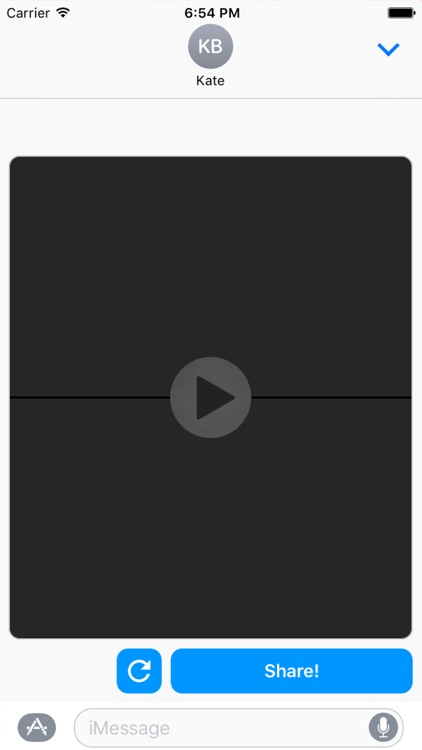The image showcases a smartphone screen interface. At the top, a status bar indicates a strong signal (full WiFi) and a fully charged battery. The resolution is displayed as 654p, and the initials "KB" are visibly encircled, possibly indicating a specific setting or notification. A blue downward arrow signifies a download or drop-down menu. The image features black edges framing a central circular play button, which is positioned above a horizontal line.

Within the interface, there are several interactive elements: 
- A blue square labeled "OIR" accompanied by a refresh button. 
- Another blue element marked "Share." 
- A square symbol with a compass icon, indicating navigation or location services.

Additional icons include an oval indicative of a message, a circle symbol for recording or voice commands (microphone), and a depiction of a smartphone. The background is predominantly grey, presenting a stark contrast to the more colorful interface elements, but it contains little other detail or visual information.